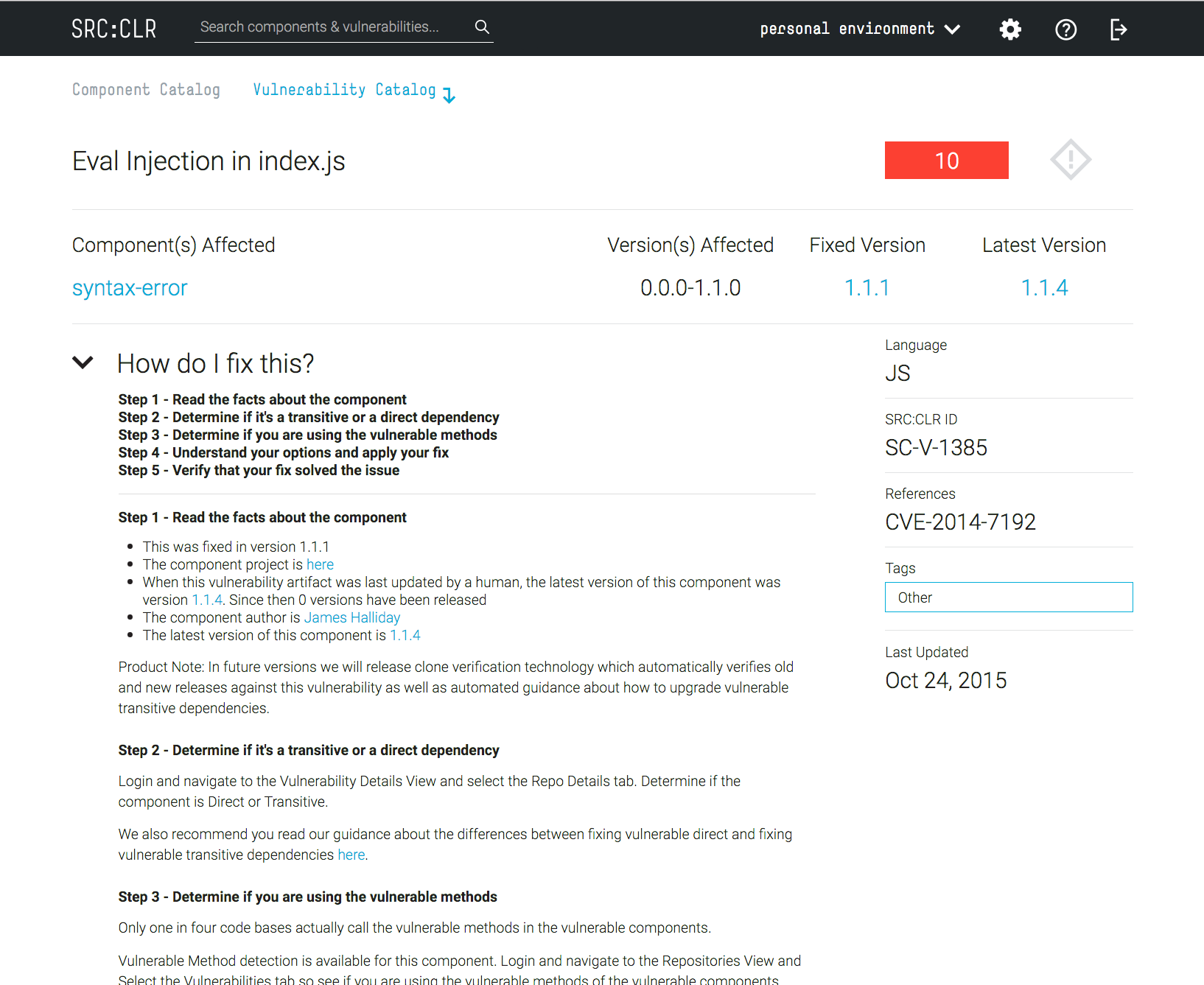### Detailed Caption

At the top of the page, there is a black border with the text "src: clr" prominently displayed. Below it, a search box allows users to enter queries with the placeholder text "Search components and vulnerabilities." Adjacent to this, on the right, there is a gear icon and a question mark enclosed in a circle, offering additional settings and help options.

Underneath, the page is divided into two main sections: "Component Catalog" and "Vulnerability Catalog," with the latter being highlighted in blue. Within this section, the header "Eval Injection in index.js" is displayed, followed by "Components Affected: Syntax Error."

The central content is a step-by-step guide to resolving the vulnerability:

1. **Read the facts about the component:**
   - This issue was fixed in version 1.1.1.
   - The latest version available of the component when the artifact was updated by a human is 1.1.4.
   - A total of zero versions have been released since then.
   - The component author is James Halliday.

2. **Determine if it's a transitive or a direct dependency:** Detailed instructions are provided.

3. **Determine if you are using the vulnerable methods:** Detailed instructions are provided.

4. **Understand your options and apply your fix:**

5. **Verify that your fix solved the issue:**

Additionally, it notes that "In future versions, we will release clone verification technology."

On the right side of the page, there is a sidebar showing the versions affected, the fixed version, and the latest version, along with additional metadata such as language, references, tags, and the last update date.